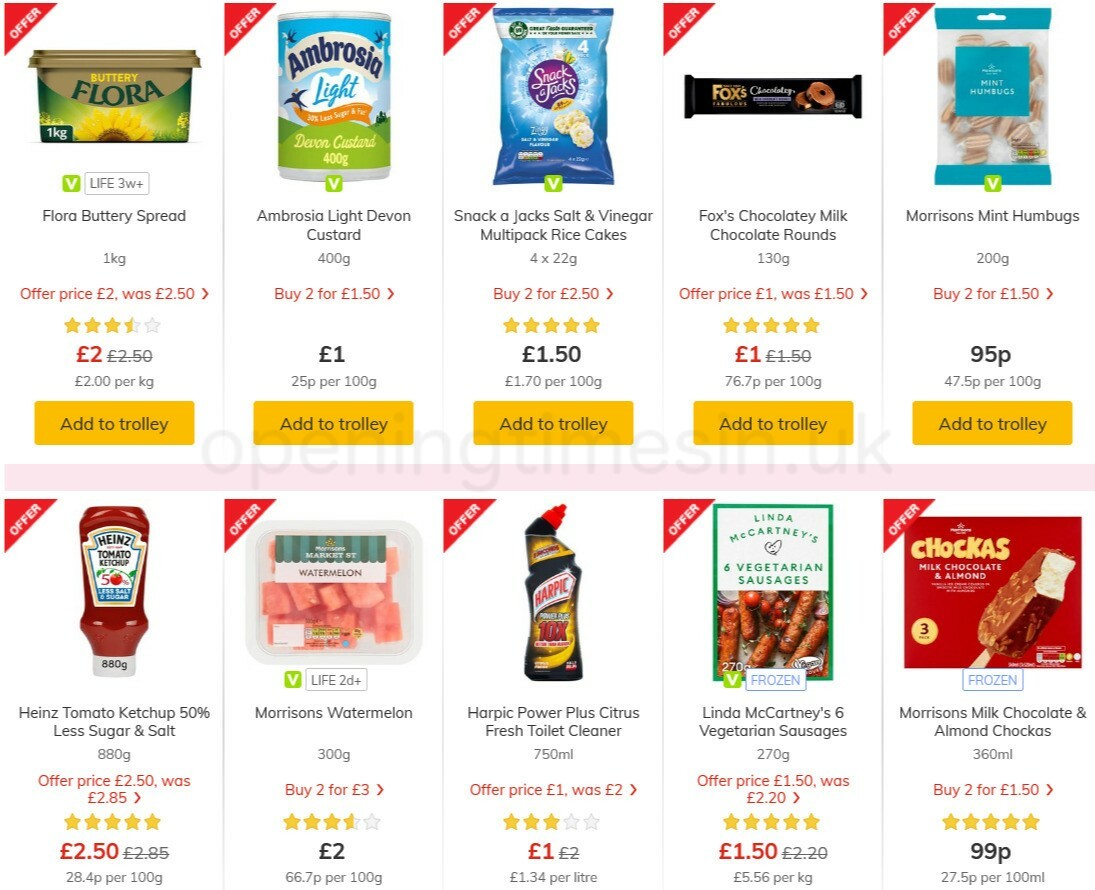A detailed screenshot showcases 10 different products available for purchase, indicating a British online grocery, given the reference to "trolley" and prices in pounds. 

1. **Buttery Flora Spread**: A 1 kilogram tub priced at £2. Ideal for adding a creamy flavor to your dishes.

2. **Ambrosia Light Devon Custard**: Available at a promotional offer of 2 packs for £1.50, perfect for a light dessert option.

3. **Snack-a-Jacks Salt and Vinegar Multi-Pack Rice Cakes**: On sale for 2 packs at £2.50, a savory snack choice.

4. **Fox's Chocolatey Milk Chocolate Brownies**: A rich and indulgent treat.

5. **Morrisons Mint Humbugs**: Priced at just 95 pence, these classic mint candies are an affordable option.

6. **Heinz Tomato Ketchup**: A healthier version with 50% less sugar and salt, perfect for those watching their intake.

7. **Morrisons Watermelon**: Fresh and juicy, a refreshing fruit option.

8. **Harpic Power Plus Citric Toilet Bowl Cleaner**: Ensures a clean and hygienic bathroom.

9. **Linda McCartney's Vegetarian Sausages**: A meat-free alternative, great for vegetarians.

10. **Morrisons Milk Chocolate and Almond Chukkas**: A delightful ice cream treat that combines creamy milk chocolate with crunchy almonds.

All these products are highlighted for their affordability and variety, appealing to a broad range of tastes and needs.